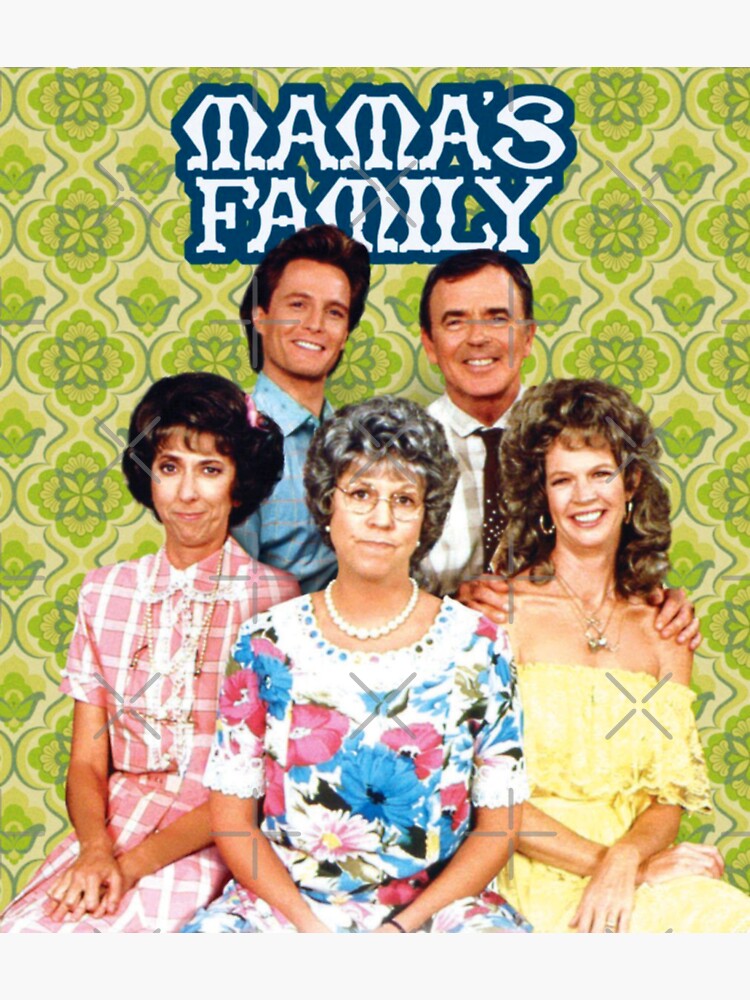The image is a promotional photo for the television show Mama's Family. The title "Mama's Family" is prominently displayed at the top in white font, surrounded by a dark teal border around each letter. The photo features five Caucasian characters against a background with a green, leaf-like, and curved pattern, which also includes a transparent watermark shaped like a cross and the letter X. In the foreground, there are three women: on the left, a brunette in a pink and white checkered dress; in the center, an older woman with curled gray hair, wearing a white pearl necklace and a purple dress adorned with blue, pink, and green flowers (identified as Vickie Lawrence, who plays the matriarch "Mama"); and on the right, a woman in a yellow dress. In the background, two smiling males are standing. All are looking towards the camera, smiling. This sitcom, believed to have aired on either NBC or ABC in the United States, depicts the matriarchal figure central to the family dynamics.